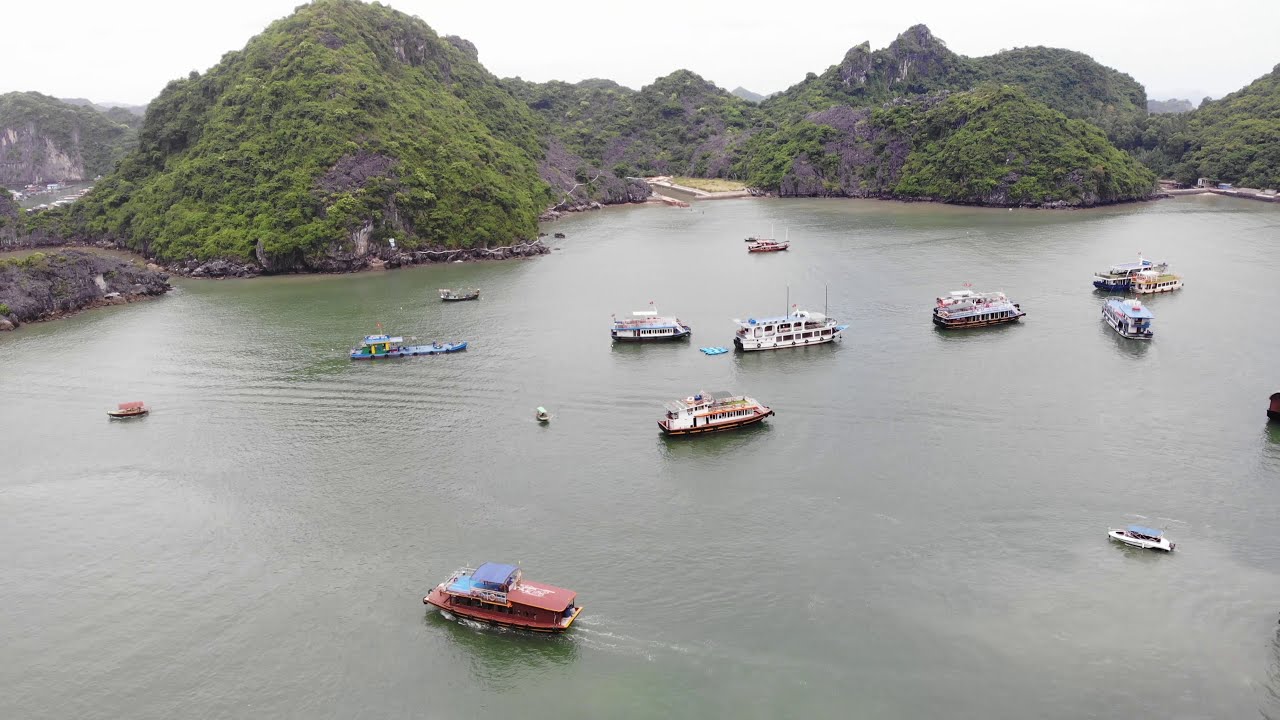In the image, an aerial shot captures a coastal scene featuring a calm body of blue and gray water, dotted with approximately fifteen boats of varying sizes and colors. Most of these vessels are square-shaped passenger boats, many of which are two-story. The boats primarily appear in white with different colored trims, such as black and orange, along with a notable red boat closest to the foreground, bearing white lettering and a blue canopy. Behind the boats, the landscape reveals multiple hills and cliffs, predominantly covered in green grass and trees, though some brown patches and rocky areas are visible. The sky above is a cloudless gray, creating a serene, muted backdrop. On the left side of the image, behind the hills, structures suggest the presence of buildings or possibly a port, indicating a populated area.